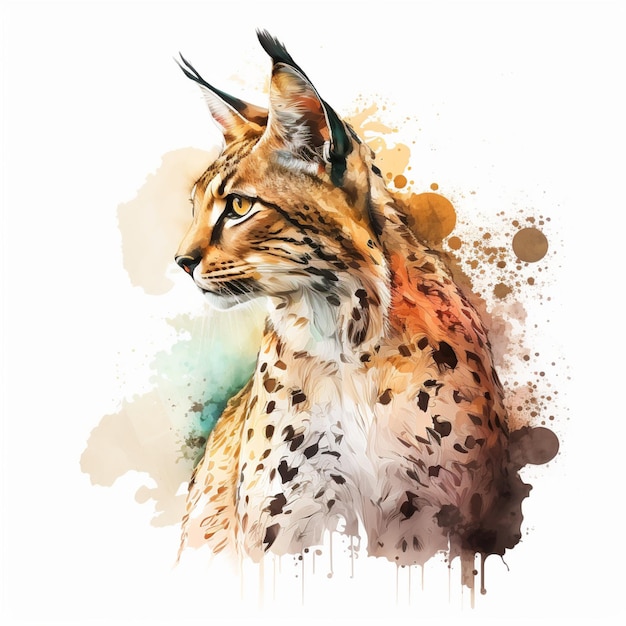This painting depicts a strikingly detailed wild cat, often identified as a bobcat or lynx, set against a minimalistic white background with abstract watercolor splotches in beige, light pink, dark and light brown, and hints of bluish-green. The artist masterfully captures the luxurious texture of the cat's fur through expressive brushstrokes, presenting a lifelike impression of the creature. The cat itself boasts a predominantly white coat sprinkled with dark spots, while the head features a captivating light brownish-gold hue. The cat's body faces forward, yet its head is turned to the left, showcasing a bright amber, almost yellow, eye that conveys a keen sense of alertness. Its large, pointed ears, topped with tufts of black fur, stand erect as if listening to its surroundings. The absence of any text allows the detailed and vibrant portrayal of the cat to take center stage in the composition.